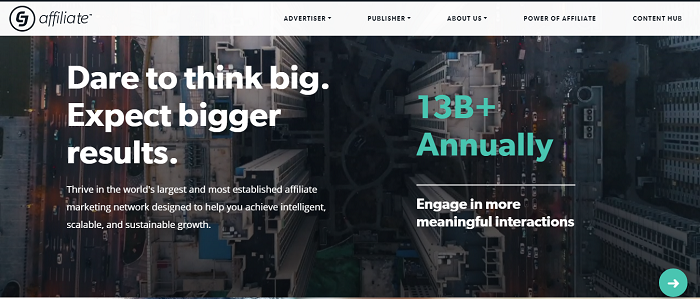This screenshot from the Affiliate website prominently features its brand slogan, "Dare to Think Bigger," accompanied by the phrase "Expect Bigger Results." Below, the under-slogan reads, "Thrive in the world's largest and most established affiliate marketing network designed to help you achieve intelligent, scalable, and sustainable growth." The website boasts an impressive annual profit of approximately $13 billion and emphasizes its commitment to engaging in meaningful conversations with its users.

At the top of the webpage, several navigation headings are visible, such as Advertiser, Publisher, About Us, Powerful Affiliate, and Content Hub. The background displays a dynamic cityscape with flowing traffic, adding a sense of movement and modernity. At the bottom, options for interacting further with the website are offered, indicating multiple layers of marketing features. This detailed screenshot encapsulates Affiliate's robust online presence and its focus on expansive, scalable growth in the affiliate marketing industry.